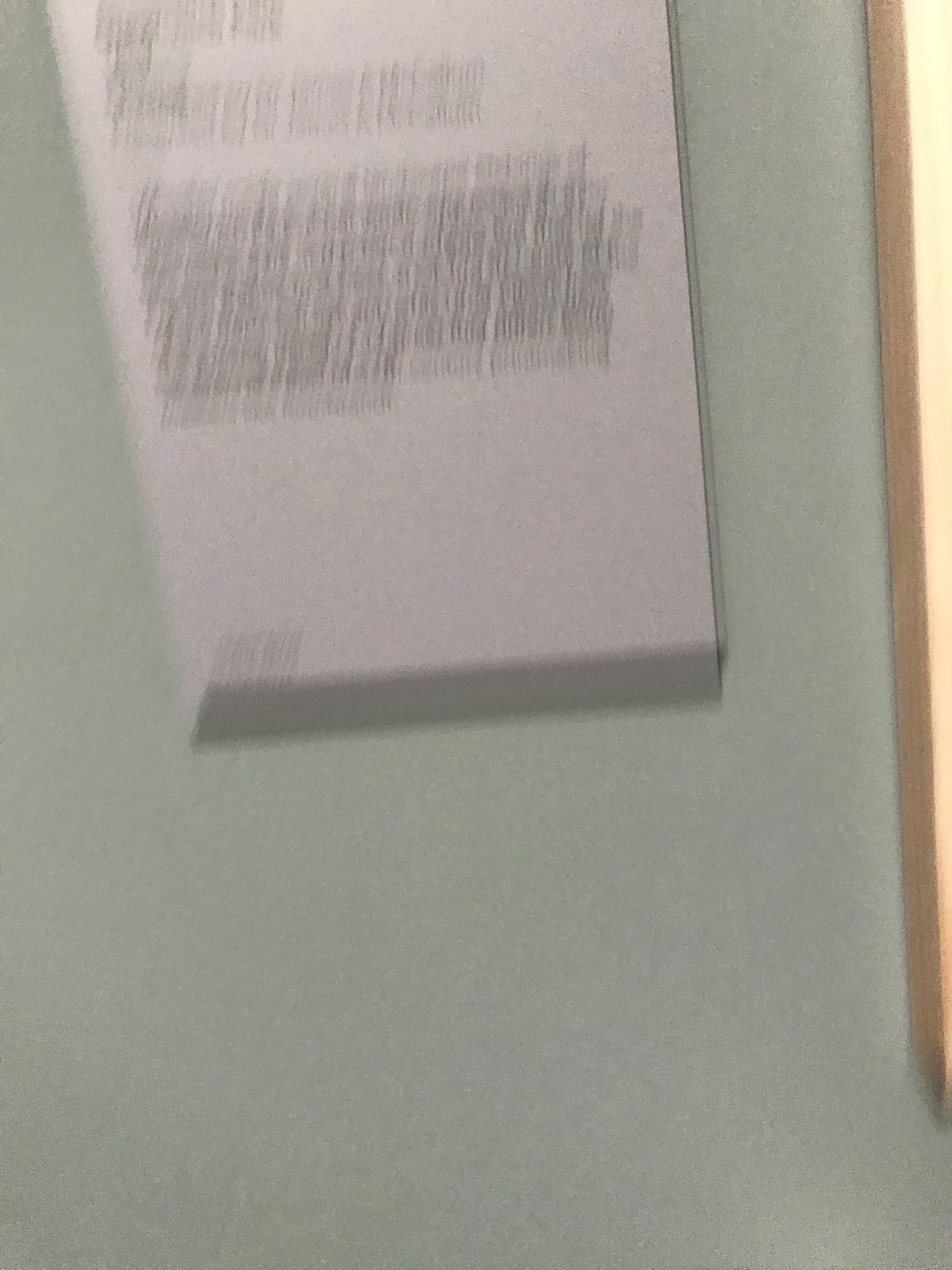The image depicts a white rectangular sign affixed to a light beige or grayish-green wall, partially obscured by motion blur. The sign displays several paragraphs of black text, though the precise content remains unreadable due to the blurriness. A wooden vertical frame, made of light blonde wood, is visible on the right side of the photograph, possibly belonging to a window or bulletin board, extending nearly to the bottom of the image. The overall scene is characterized by its out-of-focus quality, with shadows suggesting top-down lighting. The blurred text appears to be organized with sections of varying sizes, hinting at a header and subsequent detailed paragraphs.